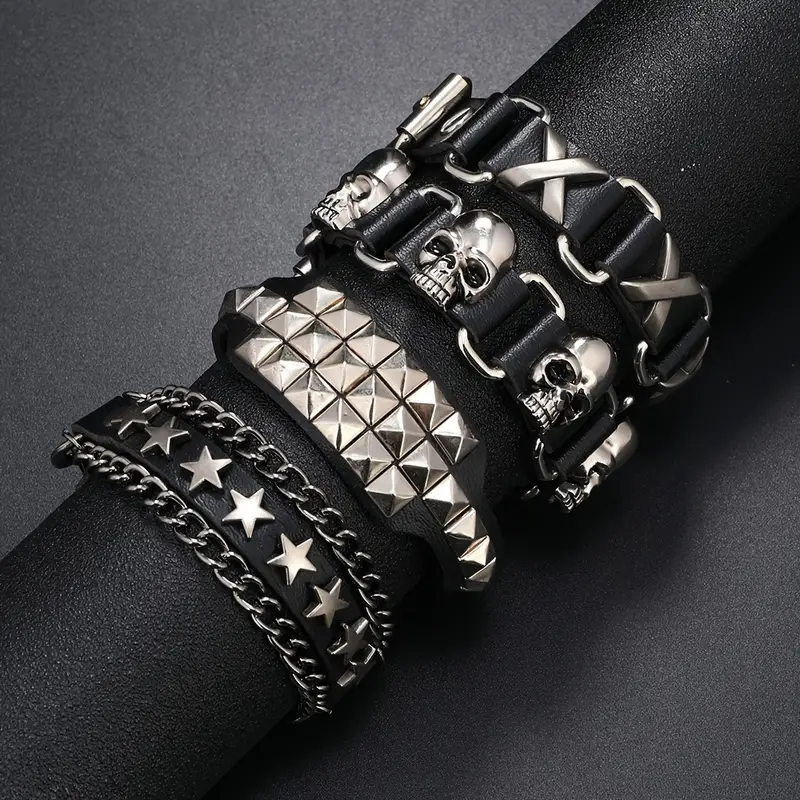In this meticulously detailed photograph, taken from above, someone's arm is adorned with four distinct black leather bracelets, each showcasing intricate silver designs. The background contrasts in shades of light to medium gray, highlighting the bracelets. The topmost bracelet features a black leather band with alternating silver crosses and chain links, exuding a bold, edgy aesthetic. Below it, the second bracelet mirrors the chain link style but stands out with its silver skulls embedded along a strip of black leather. The third bracelet breaks from the chain motif, presenting a sleek black cuff accentuated with shiny silver squares. The bottom bracelet completes the ensemble with a row of silver stars framed by a border of silver chain links along the top and bottom edges, adding a touch of celestial flair. The arm and its adornments create a striking visual juxtaposition against the textured, sandpapery gray background, enhancing each bracelet's unique design elements.